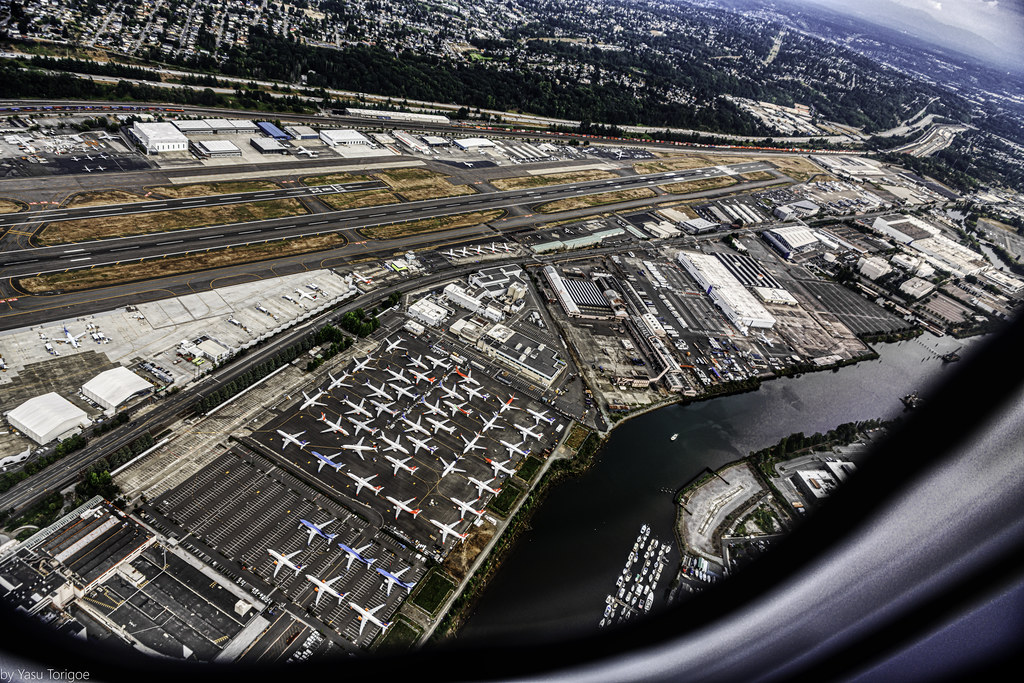This detailed color photograph, taken from the window of an airplane, offers a sweeping aerial view comprising a bustling cityscape below, partially obscured by the plane's window outline. Central to the image is an expansive airport complex with two parallel runways prominently visible, flanked by numerous gates and parking areas filled with aircraft. In the bottom left corner, there are large parking lots with tightly lined commercial airliners, approximately 30 in one lot and six in another adjacent lot. Surrounding the airport are industrial structures, buildings, and extensive roadway networks, suggesting a busy metropolitan area. A significant canal cuts through the lower right section of the image, adding depth and dimension to the landscape. The view stretches into the distance, revealing neighborhoods, tree-lined areas, and possibly a mountainous region in the far background. The photograph captures the essence of a densely populated area intertwined with natural features, housing, and significant infrastructure, emphasizing the airport's integral role within this urban setting.